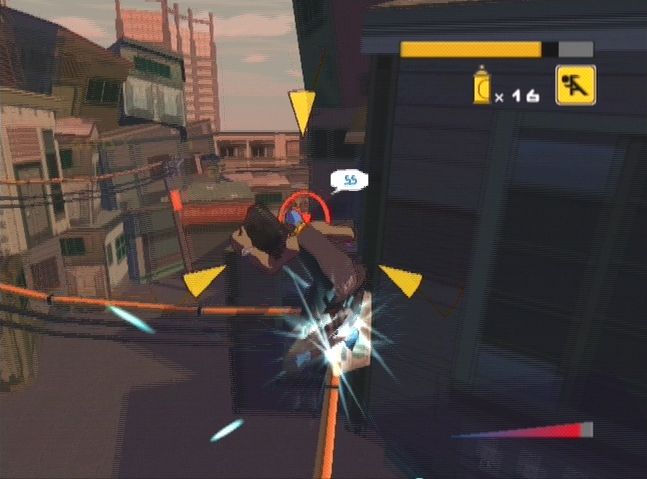The screenshot appears to be from a video game, shown in landscape orientation within a rectangular frame. The background reveals an expansive blue sky dotted with clouds. Dominating the left-hand side of the image is a dystopian cityscape, featuring a mishmash of tall, uneven buildings with skewed lines and funky angles. Interspersed among the structures are power lines, accentuating the rundown atmosphere.

The right-hand side of the screen displays an interface, possibly the game's dashboard, indicating elements relevant to the player. Featured prominently at the top is an icon of a spray can, colored orange, with the text "SPRAY CAN x1" written in white next to a thumbs-up symbol. Beside this icon is another small square, illustrating a running figure in orange.

In the center of the image, the main character is depicted with his back to the viewer. He appears to be wearing headphones and is seen grinding down a rail, presumably on a skateboard, though both the skateboard and his legs are somewhat indistinct. Highlighting the character's position are three yellow triangles, all pointing towards him. The character is also carrying a boom box on his shoulder, suggesting an urban, rebellious theme. His feet seem to emanate light, hinting at a special power or ability within the game.